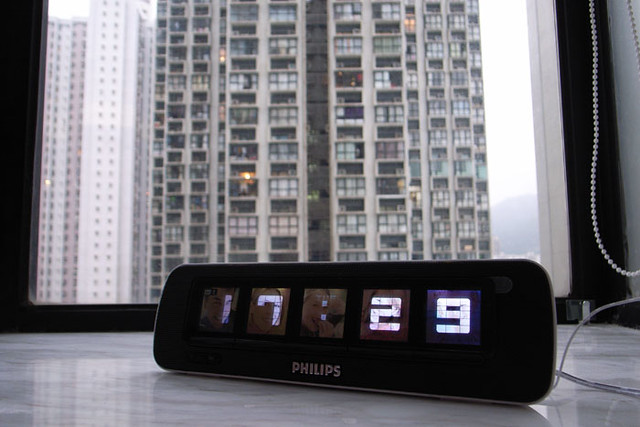The image features a sleek, modern Philips alarm clock displaying the time as 5:29 PM (1729) positioned on a granite countertop. This contemporary clock, notable for its wide yet relatively short design, rests gently on the smooth surface. In the background, a tall apartment building, rising at least 12 stories high, adds an urban touch to the scene. One can also observe the clock's wires extending off to the side and a string of beads, possibly for adjusting window blinds, subtly visible in the composition.